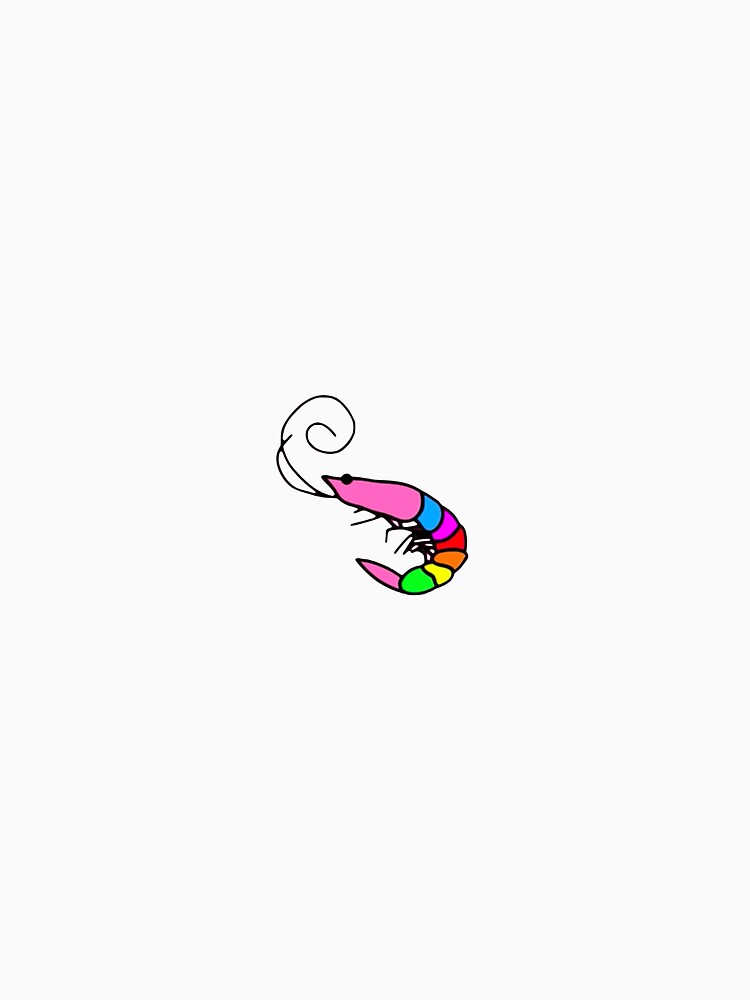The image is a vibrant, clip art style depiction of a small shrimp, prominently situated in the center of a soft cream, almost white background. The shrimp's body is vividly segmented into a spectrum of colors: the head and tail are bright pink, while the sections in between transition through turquoise blue, another shade of pink, red, orange, yellow, and bright green. The shrimp's head, positioned on the left, features a small, beady black eye. Its long, black antennae curl upwards and spiral back around, adding an animated touch to the depiction. The shrimp's body arches gracefully, with black lines indicating its legs hanging beneath the curved form. The colorful segments of its body are clearly delineated, enhancing its whimsical, rainbow-like appearance.